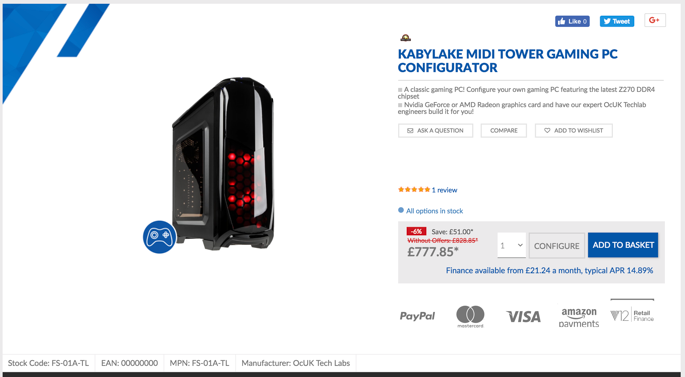**Detailed Product Description:**

This image is a screenshot showcasing a high-performance gaming PC offering. 

#### **Product Overview**
To the left, the centerpiece of the image is the **Kaby Lake Midi Tower Gaming PC Configurator**, an elegantly designed PC tower. This tower features a sleek, black case with a striking honeycomb design on the front panel, which is accentuated by a captivating red glow emanating from within. The front of the case appears to be constructed from premium glass, adding a touch of sophistication to the overall look.

#### **Product Details**
Situated on the right side is the product’s name prominently displayed in uppercase, bold, blue text: **KABY LAKE MIDI TOWER GAMING PC CONFIGURATOR**. Below this, in smaller black text, is the description: “A classic gaming PC. Configure your own gaming PC featuring the latest Z270 DDR4 chipset.” The next section elaborates on the available graphics card options, mentioning the **NVIDIA GeForce** and **AMD Radeon** graphics cards, ensuring high-quality visual performance.

#### **User Interaction**
Beneath this information, three interactive buttons are lined up horizontally: “Compare,” “Add to Wishlist,” and a third button, aiding users in making comparisons or saving the product for future consideration. This product has garnered positive feedback with one review boasting a five-star rating.

#### **Pricing and Offers**
At the bottom of the page, a grey chart outlines the pricing information. The starting price for the PC is $777.85, accompanied by a red tag displaying a discount of 6%. There is also a crossed-out price of £828.65, indicating the original cost without the discount. The text “Save £51 *” signifies additional savings. 

#### **Purchase Options**
To the right of these details, two prominent blue buttons offer direct actions for prospective buyers: “Configure” and “Add to Basket.” The image also notes financing options, stating, "Finance available for £21.24 a month with a typical APR of 14.89%."

#### **Payment Methods**
The bottom section of the image lists various payment methods including **PayPal, MasterCard, Visa, Amazon Payments,** and **V12 Retail Finance**, providing multiple convenient transaction options.

This detailed description encapsulates all facets of the product, aiming to provide potential buyers with a comprehensive insight into the Kaby Lake Midi Tower Gaming PC Configurator, its features, pricing, and purchasing options.